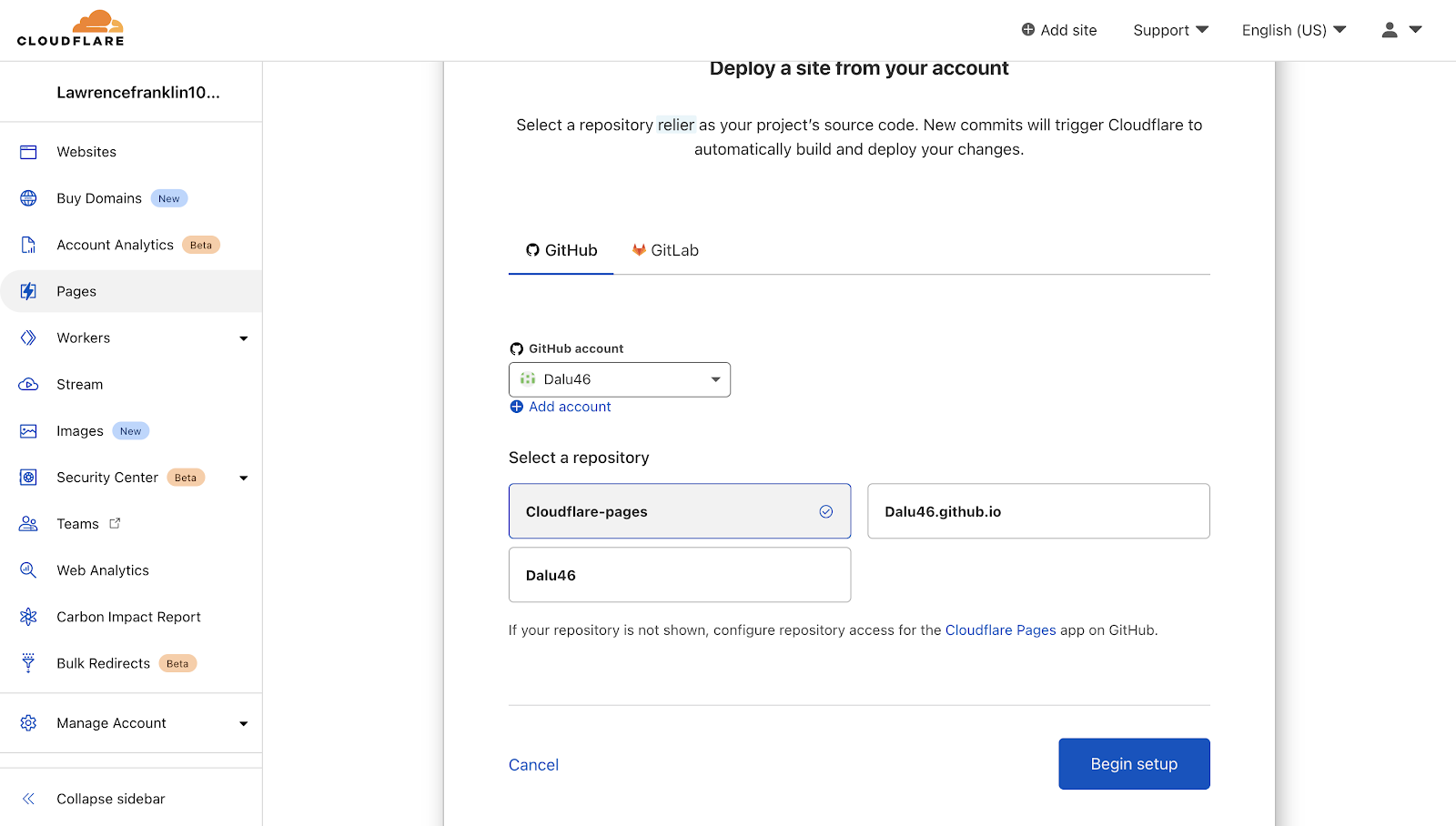This is a detailed screenshot of a CloudFlare website interface. In the upper left corner, the CloudFlare logo is prominently displayed in black font, accompanied by a small yellow cloud icon with an arrow above it. On the upper right corner, the navigation menu includes several options: "Add Site" with a plus sign, "Support" with a drop-down arrow, "English, US" with a drop-down arrow, and a silhouette of a person with another drop-down arrow next to it. The background of the website is primarily white, promoting a clean and organized look.

Along the left side of the webpage, there is a vertical menu featuring various clickable items. At the very top of this menu, it is labeled "Lawrence Franklin 10..." followed by a dividing black line. Below the line are menu options listed as: Websites, By Domains, Account Analytics, Pages, Workers, Stream, Images, Security Center, Teams, Web Analytics, Carbon Impact Report, Bulk Reports, Manage Account, and Collapse Sidebar. The "Pages" option is currently selected, evident by its slightly grayed-out appearance.

To the right of the menu, the main content area displays the "Pages" section details. The header states, "Deploy a site from your account." Beneath this, it explains that users can select a repository provider as their project source code, and new commits will trigger CloudFlare to automatically build and deploy any changes. Two provider options are listed below: GitHub and GitLab, with GitHub currently chosen.